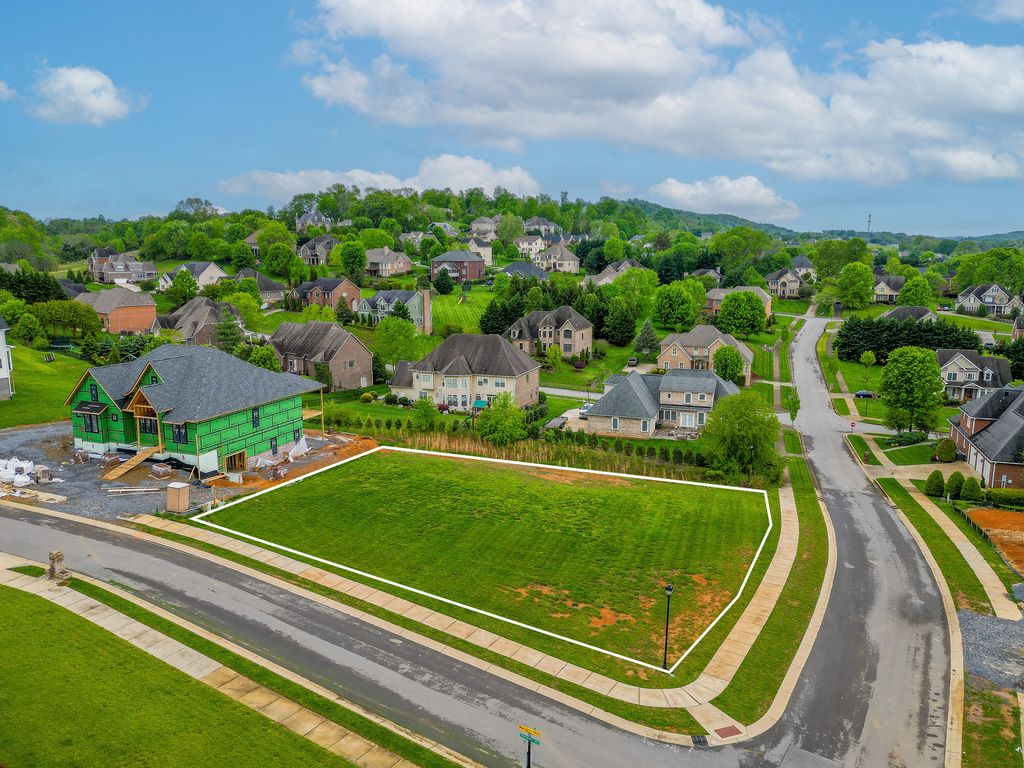This aerial photograph captures a picturesque, middle- to upper-middle-class village or neighborhood on a clear, sunny day with fluffy white clouds dotting the blue sky. The scene provides a detailed layout; multiple roads and sidewalks carve through rows of beige buildings, many adorned with gray roofs. The landscape is lush and green, with small trees scattered between the buildings. The neighborhood is framed by low hills and distant mountains, emphasizing the serene setting.

In the foreground, there's a prominent open lot dominated by a large, under-construction greenhouse. This building, wrapped in insulation with freshly shingled roofing, features a ramp leading to its entrance, suggesting active development. A big road encircles this construction site and extends into the horizon, accentuating the neighborhood's structured grid. Country roads and a V-shaped street layout add further character to the scene, portraying a well-organized and green community nestled comfortably against a verdant background.